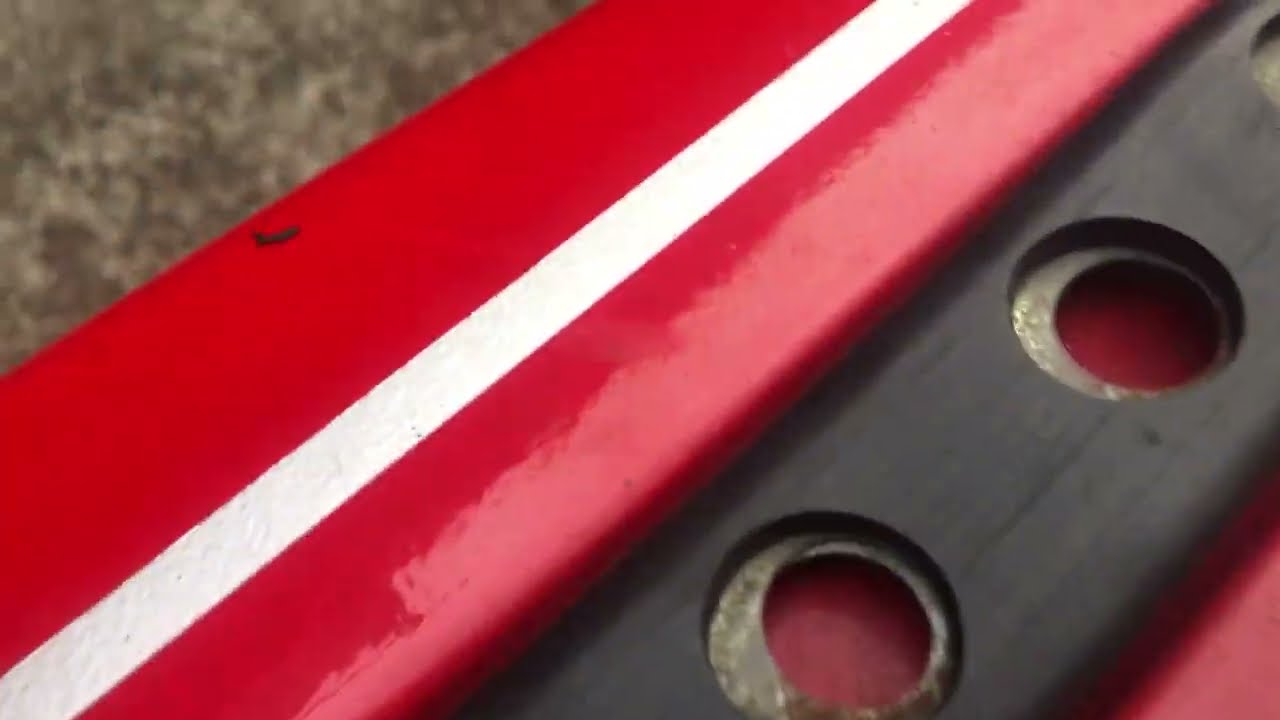The image depicts a close-up view of a machine or mechanical object, primarily featuring a deep red fiberglass or metal surface with a distinctive white stripe traversing diagonally from the lower left corner to just shy of the upper right corner. To the right of this red section lies a black segment made of a different material, perforated with holes. These holes reveal rusty golden metal circles with additional holes in their centers, giving a peek at the red layer beneath. Notably, there's a small black splotch or dot on the red material, hinting it could be a speck of dirt or a blemish. The top left corner of the image also shows a brown, sandy-like floor surface. The red section reflects light slightly, producing specular highlights that contribute to the overall detailed texture and structure of the machinery component.